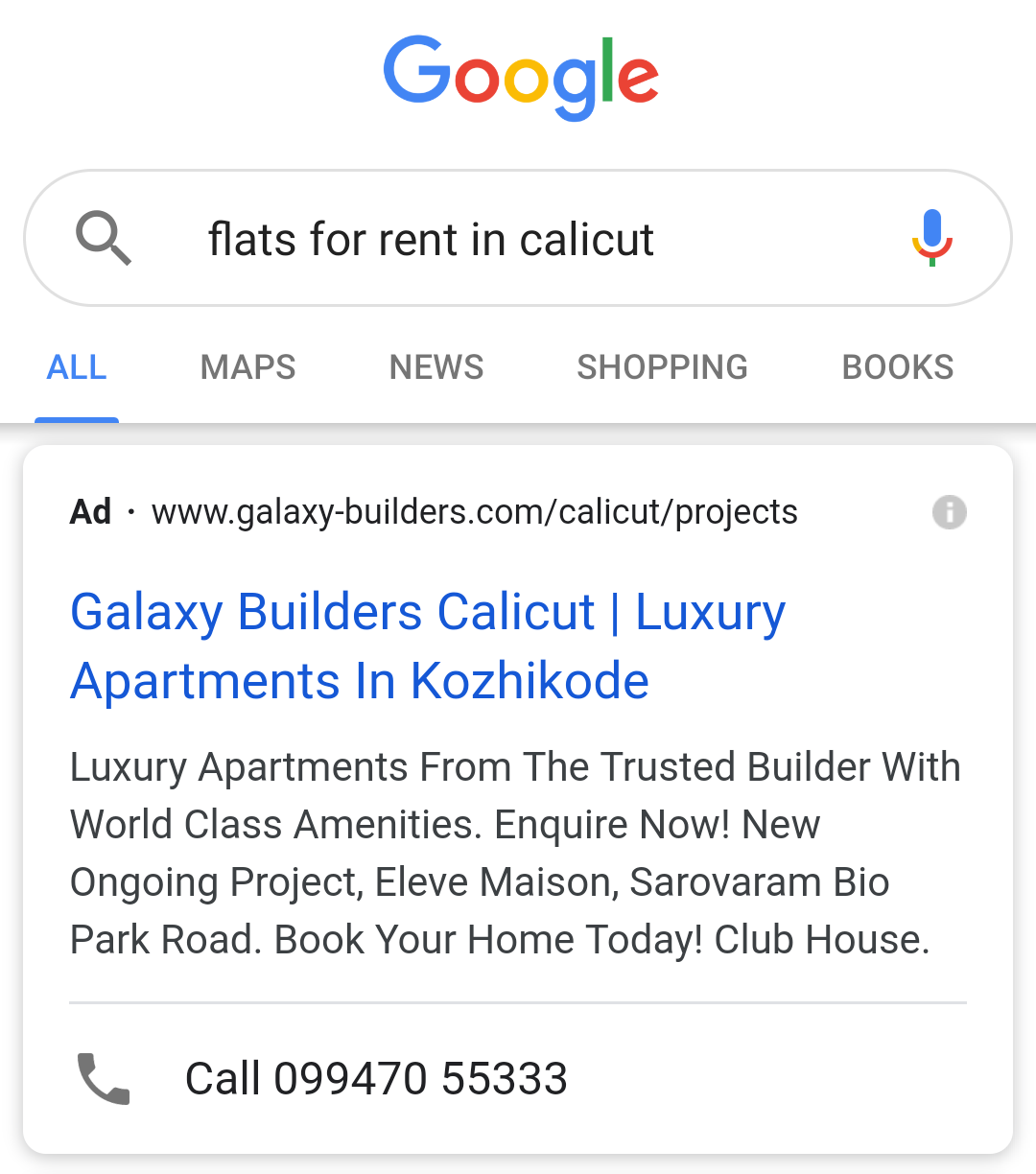The image features a clean, white background dominated by the recognizable Google logo at the top. The logo is composed of a capital blue "G," followed by a red lowercase "o," a yellow lowercase "o," a blue lowercase "g," a green lowercase "l," and a red lowercase "e." Beneath the logo is a search bar containing the phrase, "Flats for Rent in Calicut." The search bar includes a magnifying glass icon and a microphone symbol, indicative of Google's search functionalities. 

Below the search bar, there are navigational options labeled "All," "Maps," "News," "Shopping," and "Books." A pop-up box appears underneath these options. At the top of this box is the text "Ad" followed by the URL "www.galaxy-builder.com/calicut/projects" and a gray circle with a lowercase "i" inside it, signifying additional information.

The advertisement within the pop-up is highlighted in blue text, reading "Galaxy Builder, Calicut, Luxury Apartments, and Cozy Condos." Just below, in smaller black text, it states, "Luxury Apartments from the trusted builder with world-class amenities." Additional text prompts potential buyers with messages like "Inquire Now," "New Ongoing Project," "Lee Mason, Sree Bavamam Beale Park Road," "Book Your Home Today," and "Clubhouse." This text provides a detailed call to action and emphasizes the luxurious and trustworthy nature of the listed real estate project.